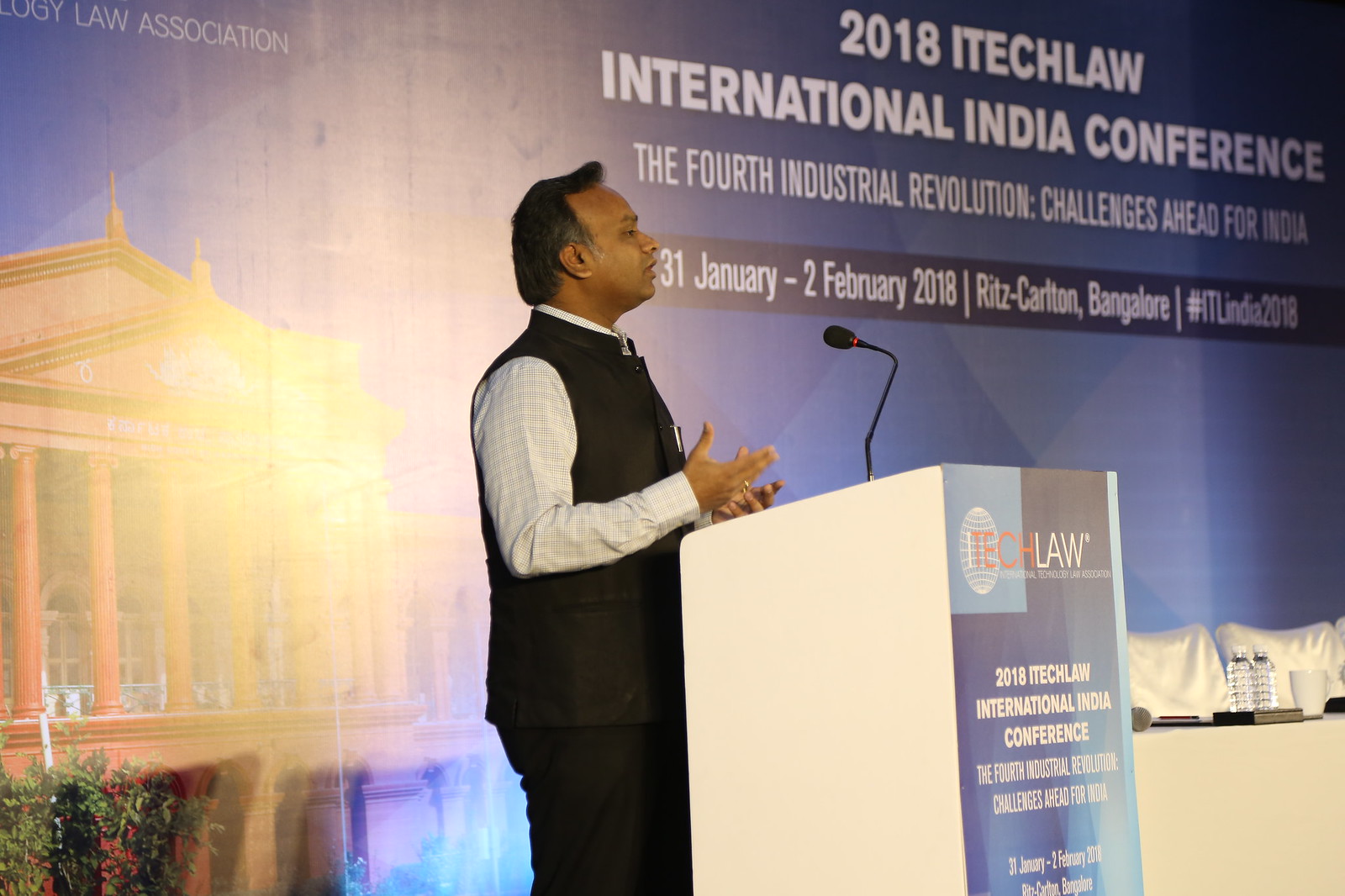In this indoor image, centered is a man standing at a white podium equipped with a microphone, seemingly delivering a speech. He is dressed in a black vest over a long-sleeved white shirt with a light grey crosshash pattern, gesticulating with his hands as he speaks. Behind him, a large banner reads "2018 I-Tech Law International India Conference, the 4th Industrial Revolution, Challenges Ahead for India, 31 January through 2 February 2018, Ritz-Carlton Bangalore, Hashtag ITL India 2018." On the podium's front, a sign reiterates the event details, highlighting its focus on the 4th Industrial Revolution. In the bottom left corner, an arrangement of flowers adds a touch of color, while to the right, a table holds several bottles of water and cups with a few chairs around it. The predominant colors in the scene include blue, white, gray, black, yellow, green, and red, and the setting suggests an ongoing conference.